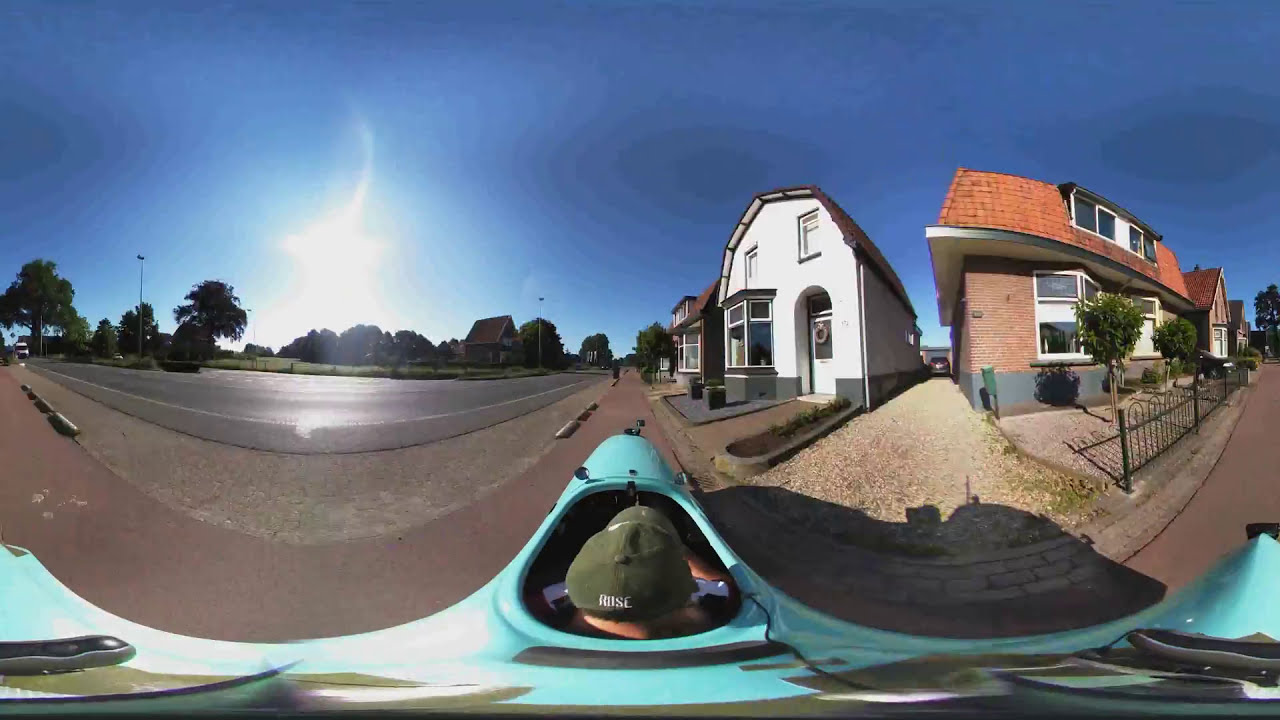This photograph, taken with a highly distorting lens, depicts a horizontal, rectangular scene that seems almost surreal due to the lens effects. The sky, a dark blue with several oversaturated hotspots, indicates a setting sun and contributes to the image's unusual lighting. Along the horizon, trees delineate a paved road that curves gently, leading the viewer's eye.

On the right side of the image, there are two distinct buildings. The first is a white house, barn-shaped, featuring a window box and partially obscured by a wrought iron fence. To its right, a larger red brick building with an expansive, unusual roof suggests it could be an apartment building or a set of condos.

In the bottom third of the image, central and distorted by the lens, appears a figure wearing a baseball cap, seemingly seated in a blue, single-passenger vehicle or possibly a kayak, adding to the overall enigma of the scene. This vehicle is stretched and skewed, complementing the surreal quality imparted by the lens. The background includes a lot or park area to one side, while variously styled buildings sit on the other side, enhancing the juxtaposition of elements within the photograph.